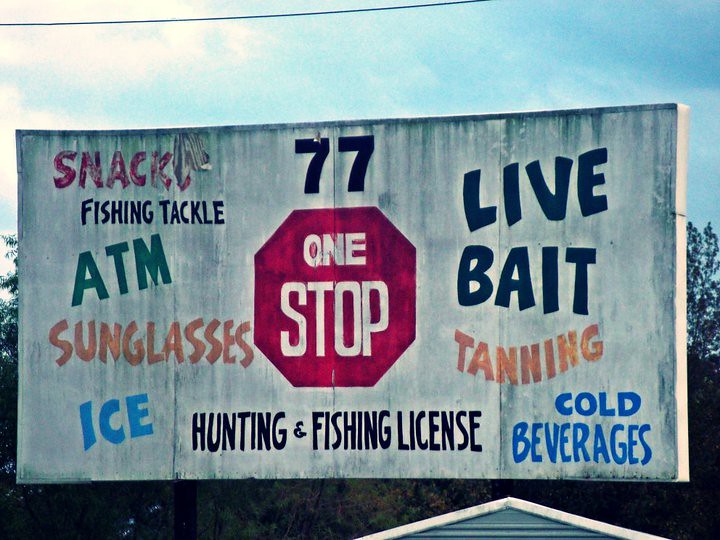This is an image of a weathered, hand-painted roadside sign, which evokes the charm of a small town roadside stop. The photograph is heavily filtered with a blue tint, giving the entire scene a cool hue. The sign itself features a prominent red stop sign in the center with the words "This is one stop" inscribed above it in black, followed by the number "77."

The text on the sign is color-coded and diverse, providing an array of services offered at this stop:
- Above the red stop sign: "77" in black.
- Below the stop sign: "Hunting and Fishing License" in black.
- To the right: "Live Bait" in black, "Tanning" in orange, and "Cold Beverages” in blue.
- To the left: "Snacks" in red, "Fishing Tackle" in black, "ATM" in green, "Sunglasses" in orange, and "Ice" in blue.

The sign appears worn and dirty, suggesting it has endured the elements for years. Beneath the sign, the peak of a small house or building is faintly visible, framed by a backdrop of trees. The sky above is partially cloudy, and a power line runs overhead, further enhancing the rural ambiance. The photograph is tightly cropped, focusing intently on the sign and its immediate surroundings.